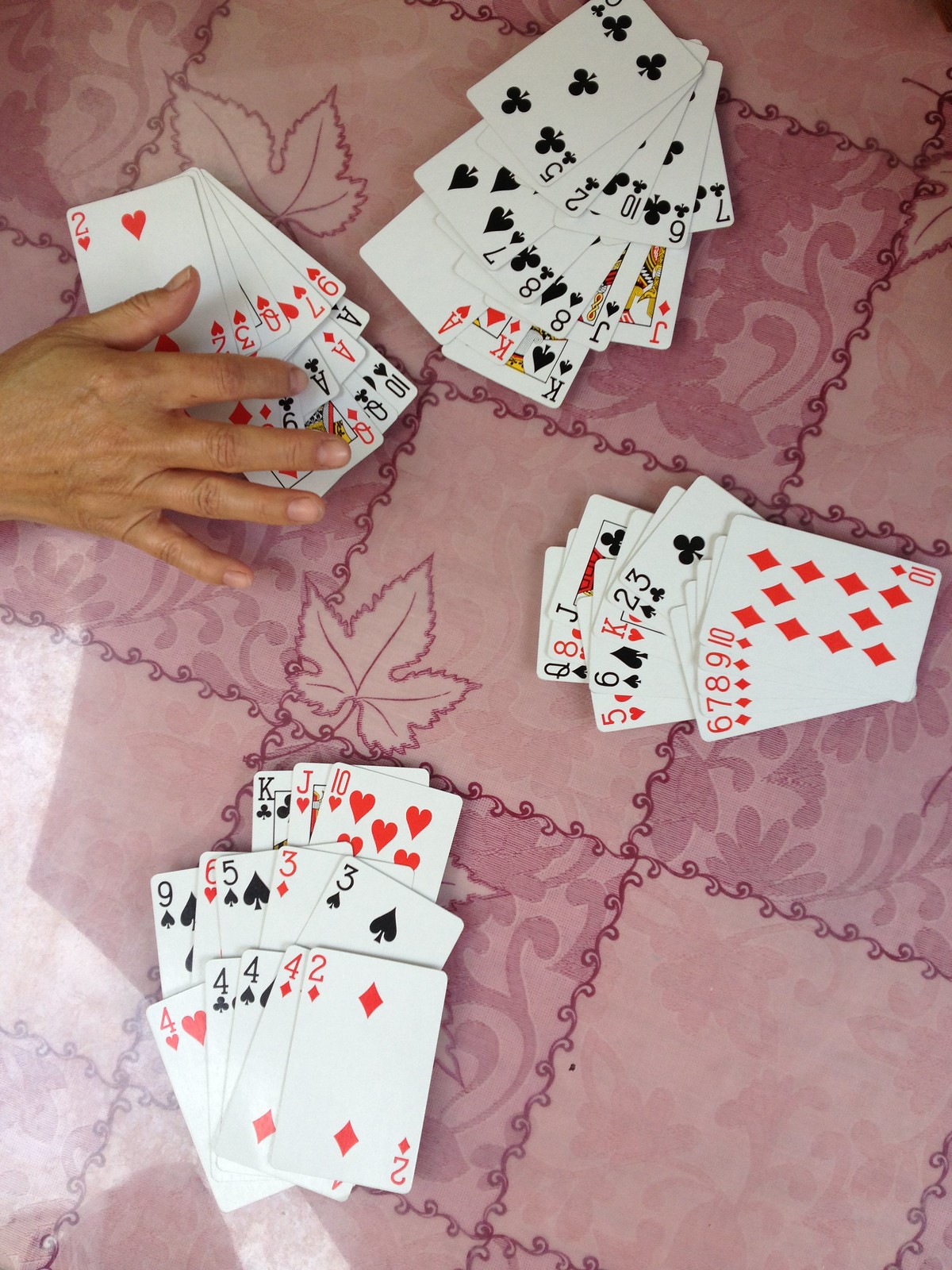This photograph captures an overhead view of a tabletop adorned with a pink and mauve patchwork-style tablecloth. The intricate tablecloth features a rich violet border that elegantly divides each patch into distinct squares. Some of these squares showcase delicate shadow floral designs, while one displays a violet-outlined maple leaf in the left-hand corner. Other squares are adorned with scroll-like floral patterns, adding to the overall enchanting aesthetic.

In the top left corner of the image, a fair-skinned right hand hovers purposefully over a set of playing cards. The cards themselves, a mix of black and white, are arranged in hands, suggesting an ongoing card game involving four players. Scattered across the tablecloth, the cards are organized into three rows per hand: the top row with three cards per hand, the middle row with five cards, and the bottom row also with five cards. The positions and orientations of the cards hint at a lively and engaging game in progress, set against the backdrop of the beautifully designed tablecloth.